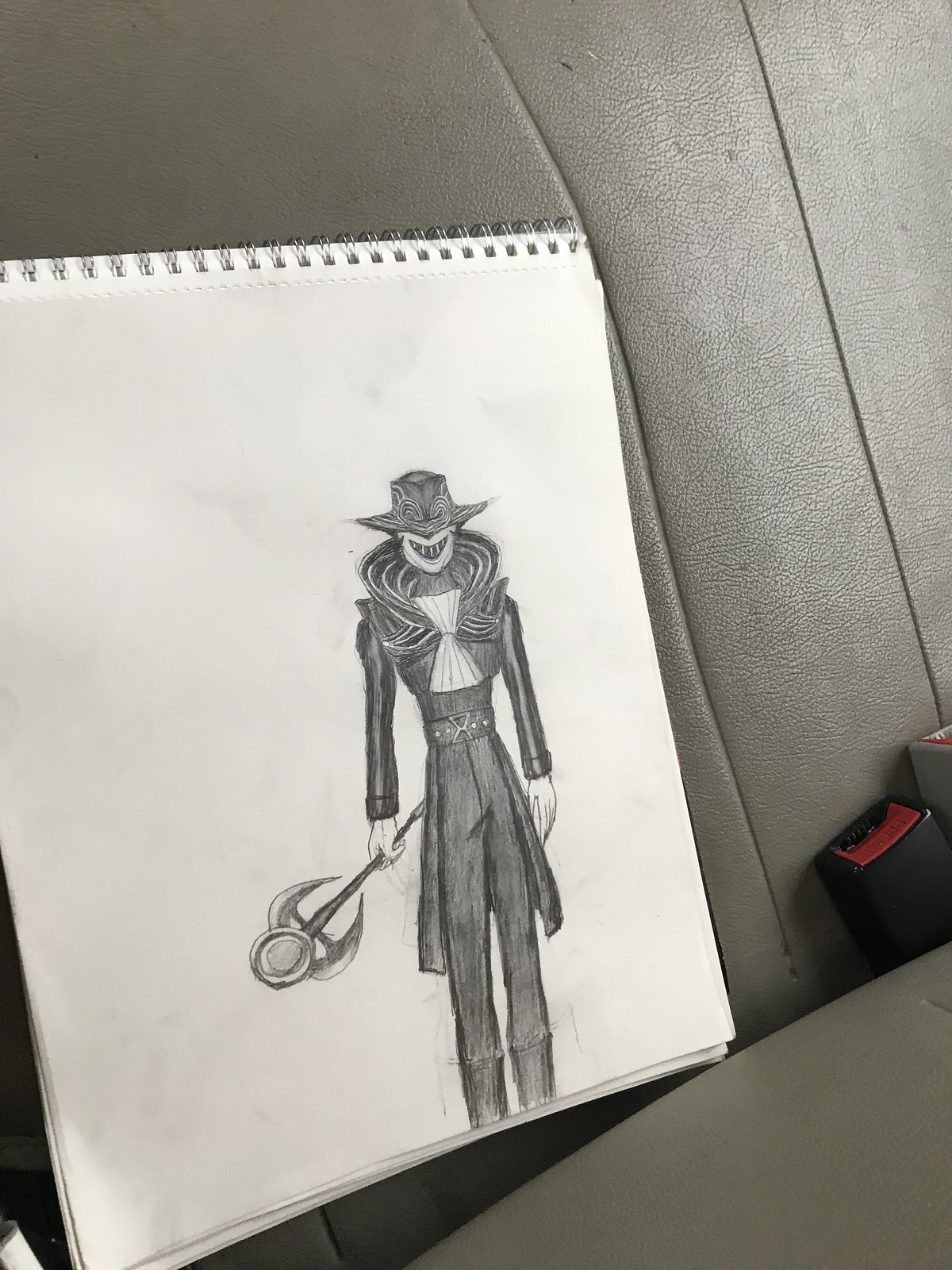This detailed photograph captures an artist's sketchbook, bound at the top, resting on the leather seat of a car. The seat belt buckle parts are partially visible, enhancing the setting of the shot. The sketch, meticulously drawn with either a pencil or black colored pencil, depicts a whimsical figure reminiscent of a joker or circus jester. The character, dressed in a hat that obscures their eyes, wears an exaggeratedly large smile and a prominently curved collar. They brandish a unique saber, characterized by a circular hilt flanked by two curved extensions, adding to the enigmatic aura of the artwork.